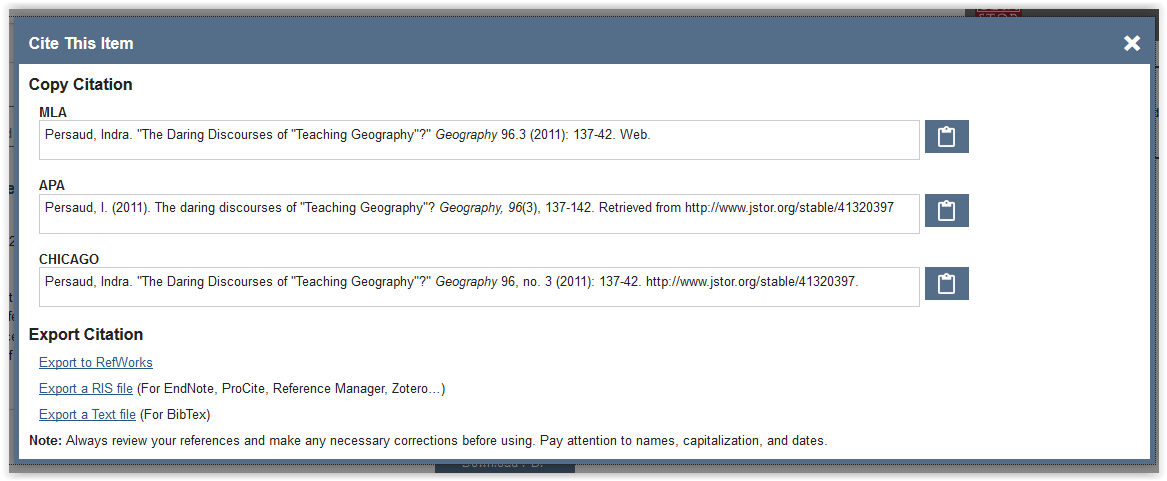This image is a screenshot of a citation tool interface. The outer border of the main text box is a dark blue, framing the section where users are prompted to "Cite this item," with the prompt text itself in crisp white. The background within this section is a clean white, providing a stark contrast to the primarily black text. However, some text elements appear as links, marked by their blue color and underlining, suggesting interactivity.

At the top of this white-background section, the words "Copy citation" are prominently displayed as a title. Below this title, three popular citation styles are listed: MLA, APA, and Chicago. Each style is accompanied by a respective text box containing a pre-formatted citation, making it easy for users to select the appropriate style for their needs. Adjacent to each text box is a blue rectangle icon that appears to depict a white clipboard, suggesting functionality for copying the citation to the user's clipboard.

Beneath the citation examples, there is an additional section labeled "Export citation," indicating further options for users to manage their citations, possibly allowing for downloads or different formats. This structured and user-friendly interface is designed to streamline the citation process for academic or research work.